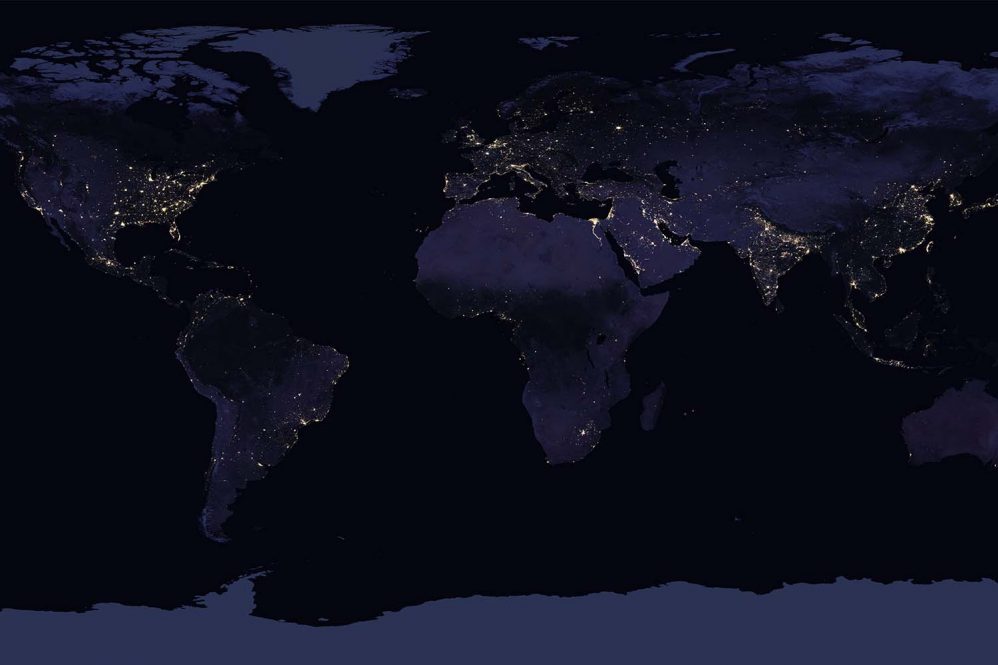This image is a detailed view of a flat world map, stretched out from west to east. The map is predominantly dark, with the waters depicted in deep shades of black and dark blue, creating a contrast against the landmasses, which are illustrated in dark charcoal hues shaded with light gray. Throughout the continents, numerous light specks in yellow are scattered, which appear to highlight densely populated areas or regions with significant electricity use. The highest concentrations of these light specks are found in the United States, parts of South America, the right side of China, and European countries, extending into the regions of Africa and the Middle East.

The background of the map incorporates purple tones alongside the dark blue, enhancing the overall geological appearance. The visual effect of these hues suggests an almost nighttime view of Earth, where the illuminated spots signify human activity amidst the darkened world. The flat representation on a rectangular canvas hints at the spherical nature of the Earth, portraying it in a two-dimensional manner that captures and merges the global perspective in one expansive image.

Additionally, the water shapes on the map somewhat resemble dynamic splashes or stirred-up mounds, further adding depth to the visual representation and suggesting the continuous and unending motion of the world's oceans. This amalgamation of darkness, light specks, and dynamic water shapes offers a vivid and insightful portrayal of the Earth's geography under a nocturnal theme.